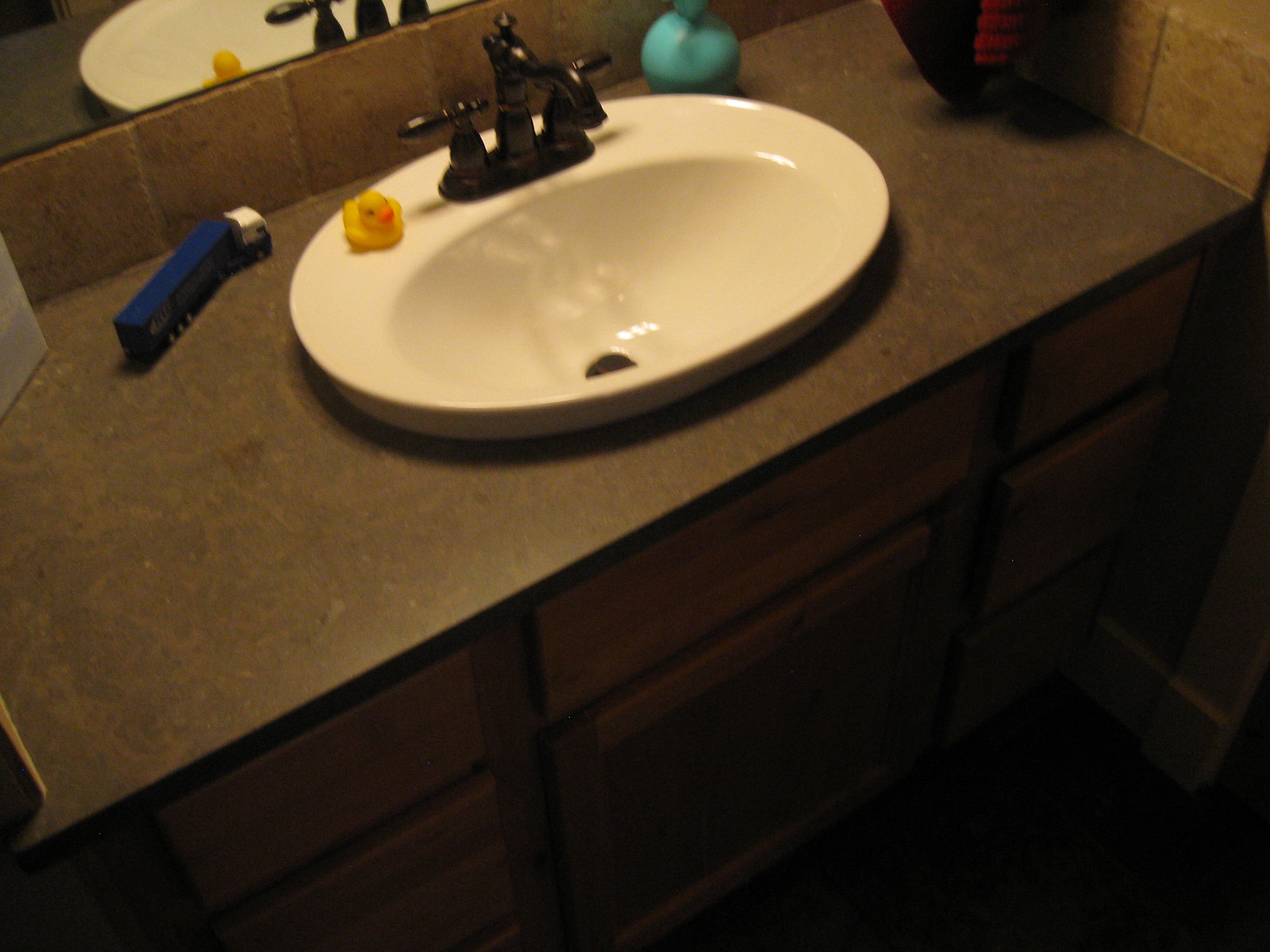This image showcases a well-decorated bathroom with a modern aesthetic. Dominating the lower part of the scene is a dark-colored wall against which a wooden vanity with three drawers—two smaller, one larger—is set. The countertop atop the vanity boasts a dark gray hue, providing a stark but elegant contrast to the wood. 

A bright blue truck with a white cab is charmingly placed on the counter. The sink basin is white, featuring black taps for a sleek look. On the left side of the sink, a yellow duck adds a playful touch. The right side of the counter holds two objects: one light yellow and another vividly red. 

Hanging neatly alongside is a light brown towel, emphasizing the natural tones in the room. Above the sink, a mirror reflects the sink area, including the duck, the basin, the towel, the countertop, and the taps, enhancing the sense of space and adding to the room's functional beauty.